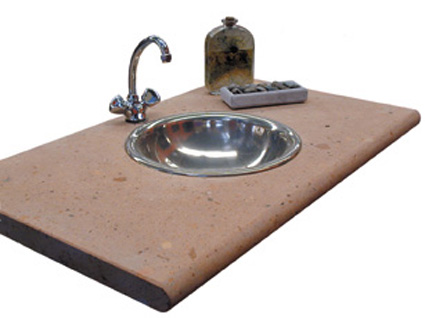This image features a small, unattached sink set up against an entirely white background, likely a mock-up for a website or catalog. The countertop is a pinkish-tan sandstone, flecked with bits of color, which contrasts subtly with the sleek, metallic sink bowl that closely resembles a silver mixing bowl. The faucet, a simple and delicate hook design, is accompanied by two handles on either side for hot and cold water control. In the backdrop, miscellaneous items such as a bottle and a collection of rocks in a concrete rectangular bowl add a touch of realism to the otherwise sterile setting.